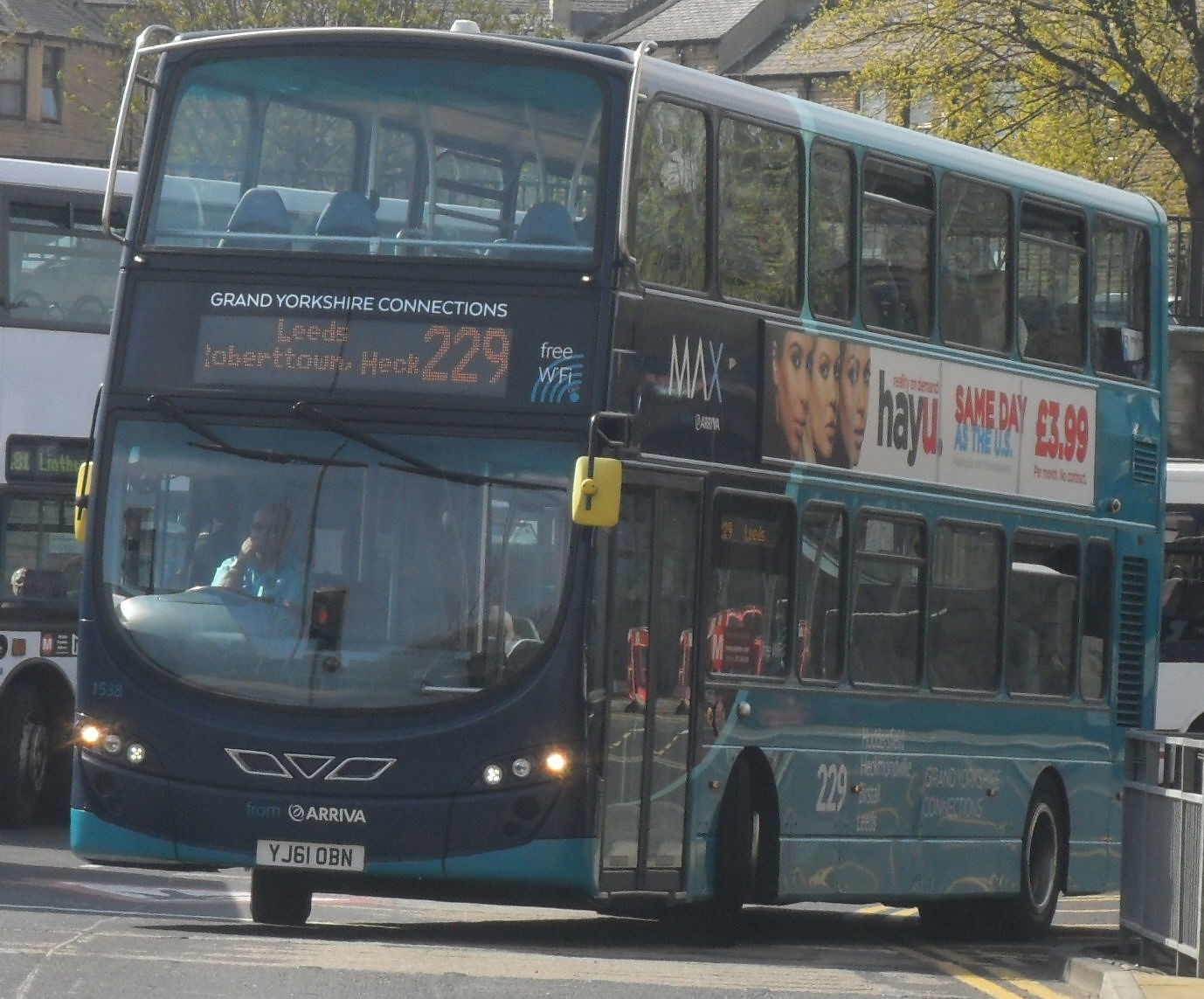A modern teal and blue double-decker bus dominates the frame, poised to move, with its wheels turned to the right. The bus features a black front and is adorned with an LED screen above the windshield displaying "Leeds, Overtown, HEC 229, Grand Yorkshire Connections," along with a free Wi-Fi symbol. The bus, captured in bright daylight, bears an advertisement banner between its levels for HAYU, promoting €3.99 per month with no contracts. The driver is positioned on the left-hand side, and behind the bus are partially obscured houses and other buses. To the right of the road, a gray steel fencing area is visible, along with trees and a substantial building, possibly a college.